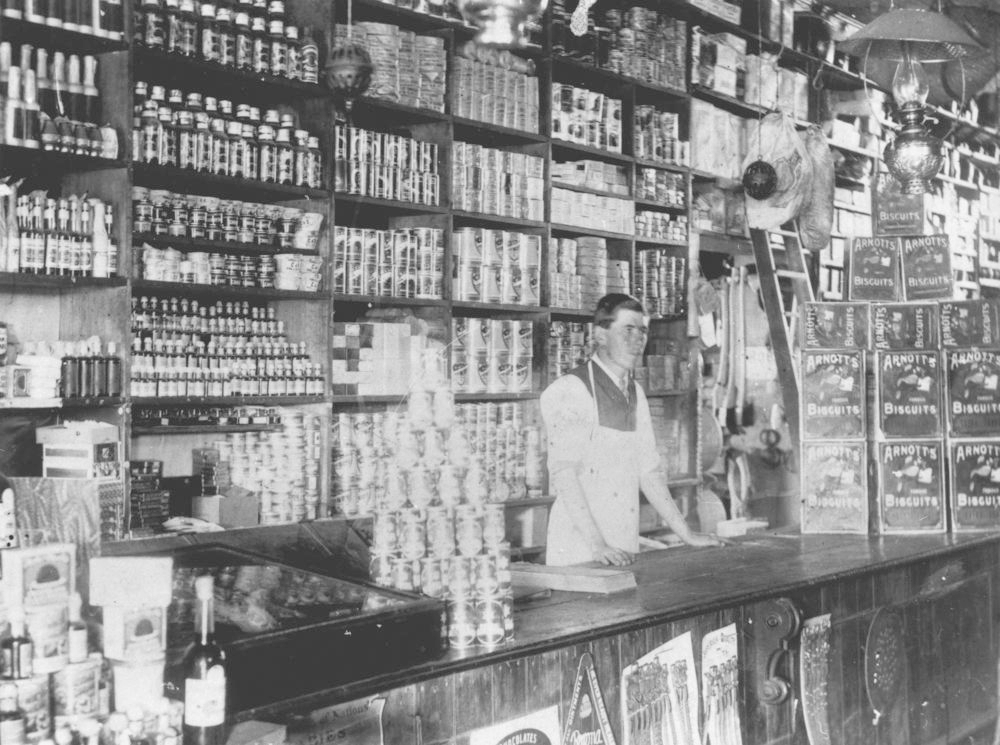This vintage black-and-white photograph captures the interior of an old mom-and-pop general store, with its quaint, bustling charm. The image is slightly blurry but strikingly evocative. Central to the frame is a young man, possibly the shopkeeper, standing behind a counter laden with various products—bottles, cans, and boxes. He has short-cropped hair, wears a white apron over a dark vest and white shirt with puffy sleeves, and a partially visible tie. His hands rest on the counter as he gazes off to the right, embodying a moment of quiet reflection in the midst of his work.

Directly behind him, shelves are densely packed with an assortment of items ranging from bottles and cans of various sizes to boxes of biscuits. On the far right, large boxes labeled "Arnott's Biscuits" are prominently stacked. A ladder leans against the shelves, partially obscured by the boxes. Additional details include the presence of newspaper clippings pinned to the front of the counter and a glass case with more items atop it, adding to the nostalgic ambiance of the store. The blend of soap, ketchup, and biscuit boxes, among other goods, enhances the sense of a diverse and well-stocked general store, capturing a slice of everyday life from a bygone era.